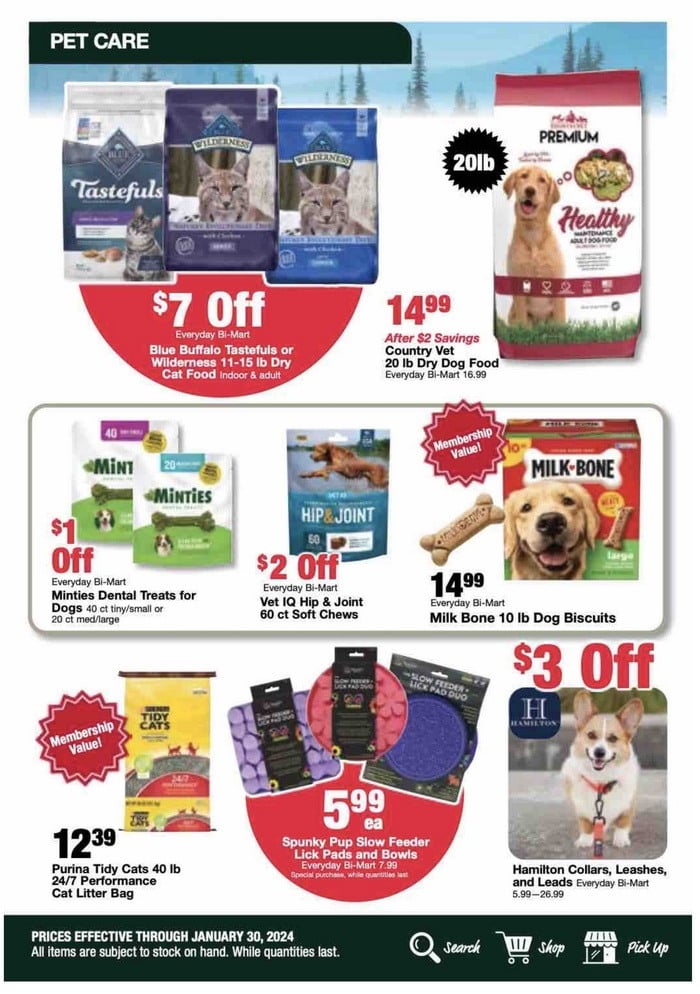This image is a detailed screenshot from a sale page on a pet care website. While the store's name isn't visible, the familiar pet care theme is clear from the content displayed. The backdrop is predominantly white, providing a clean and simple canvas for the elements on the page.

In the upper left-hand corner, "PET CARE" is boldly written in capital letters across a black rectangle, with white letters standing out for high visibility. At the top of the page, there is a small sliver of an image or a realistic drawing featuring shades of blue, depicting a mountain range and the tops of towering pine trees.

Various pet products are showcased, all advertised as being on sale. On the upper left, the Blue Buffalo Tastefuls brand is featured prominently with three images of the packaging. Two of these packages display a large gray dog, likely resembling a sheepdog.

To the right, there’s another brand which has packaging in white, featuring a light golden brown dog, possibly a golden retriever. In the central section, there are three products lined side by side. The first is called Minties, with distinctive white and green packaging, and a noticeable green bone, reminiscent of a soup bone.

The lower right-hand section grabs attention with a large red text advertising "Three Dollars Off." Beneath this, there is an adorable image of a small dog with mostly white fur, highlighted with light brown ears and head fur.

At the very bottom of the page, a black border contains a message in white text that reads, "Prices effective through January 30th, 2024." On the right side of the page, three white icons represent search, shop, and pickup options, facilitating user navigation.